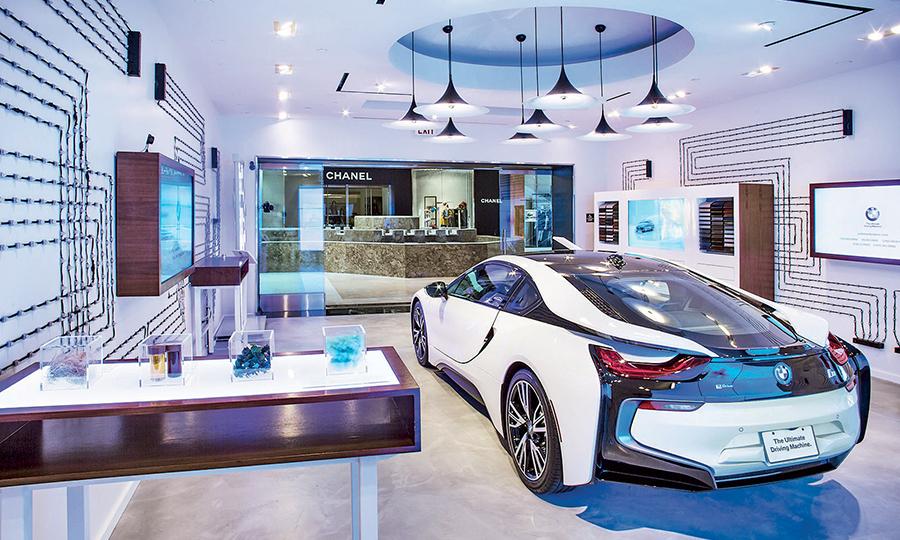This color photograph depicts the sleek, modern showroom of what is presumably a BMW store. Prominently featured in the image is a futuristic-looking, black and white BMW sports car seen from the back. The car proudly displays the iconic BMW logo and a license plate that reads "The Ultimate Driving Machine." The showroom, predominantly white, is accented with brown tables and shelves. Hanging above the car is a striking, modern light fixture with nine pendant lights arranged in a circular pattern.

The transparent glass front of the showroom opens into a shopping mall where a Chanel store is clearly visible in the background. The showroom features intricate wall designs that resemble circuit board lines, adding to the high-tech ambiance. To the left, a wooden box extends from the wall, showcasing four glass cubes in a row; these contain various colorful materials, including rainbow-like elements, gold and purple cylinders, and teal-blue crystal structures. The floor is a sleek, marble-like gray, complementing the showroom's ultra-modern aesthetic. Additional screens on the wall display the BMW logo, reinforcing the brand’s presence in this sophisticated space.